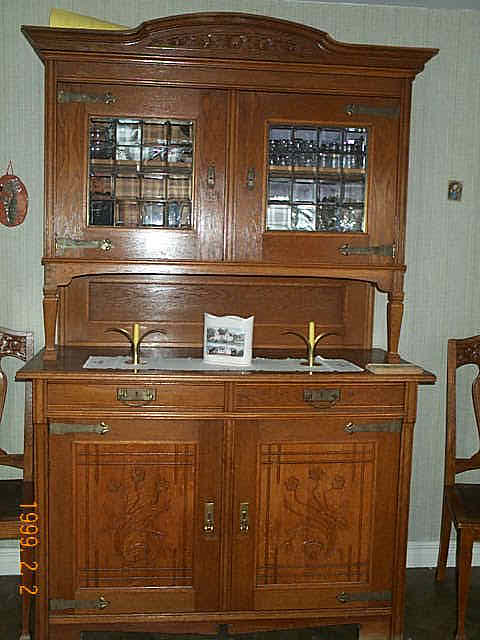The photograph, dated February 2, 1999, depicts a warmly lit indoor scene, likely within someone's home. Dominating the image is an ornate, antique wooden credenza positioned against a beige, wallpapered wall. The credenza, crafted from rich brown wood, features intricate gold-colored latches and a variety of compartments. At the very top, the credenza sports drawers and an open shelf that displays glass items, possibly glasses or cups. Beneath this, a smaller opening houses two candle holders and a framed picture. The lower section includes two central drawers flanked by two solid wood cabinet doors. Adding to the decor are wooden chairs placed on either side of the credenza and ornaments hanging on the wall. Additionally, a yellow object is visible atop the credenza. The photograph’s nostalgic aura is accentuated by a bottom left-hand corner date stamp, clearly marking a moment in time from over two decades ago.